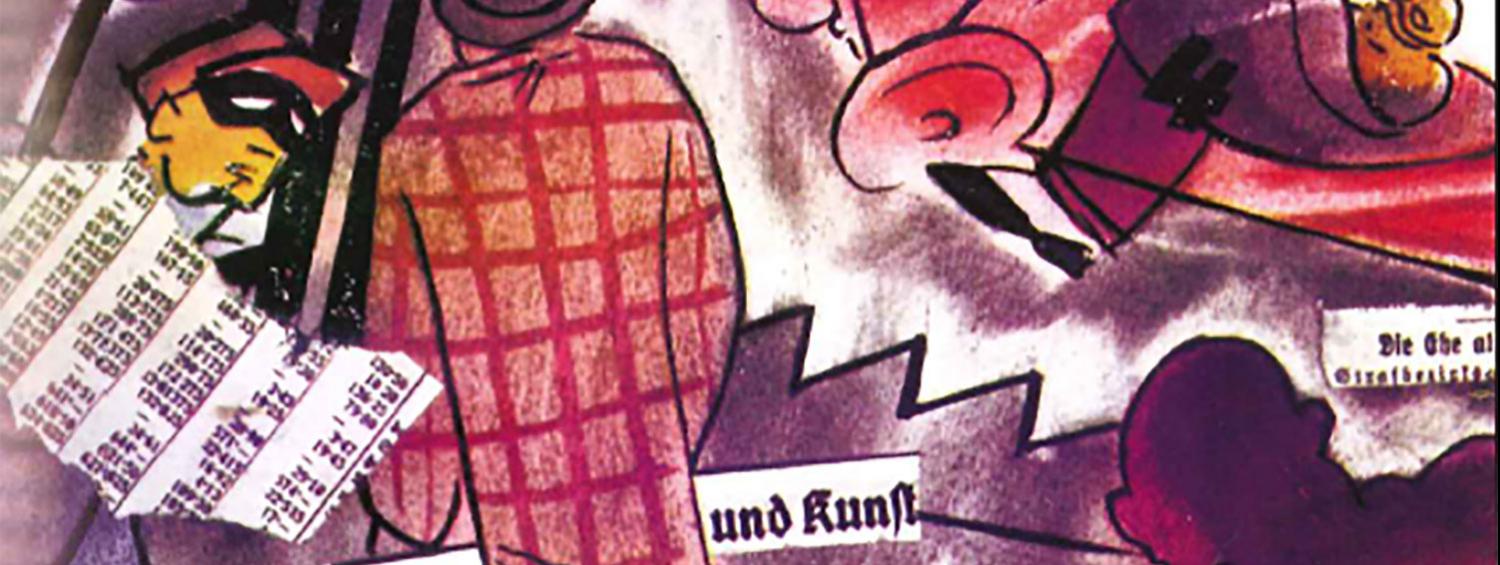The image is a vibrant, abstract collage that combines painted elements with cartoon-type characters and newspaper cutouts. Dominated by purples and pinks, the artwork features a man in the upper left corner with a yellowish face, a pink hat, and a black mask over his eyes, partially obscured by a strip of foreign-language newspaper. To the center-right of the composition stands another figure, shown from behind, wearing a partial, red-and-pink checkered coat and a purple hat. This person appears to be facing away, furthering the sense of mystery. Near the lower right corner, the back view of a man's head and muscly torso are rendered entirely in purple. Scattered across the piece are three distinct newspaper clippings, positioned on the left side, the middle bottom, and the right towards the bottom. Additionally, a red vehicle with red tires appears in the lower portion with a leg protruding out the side, adding to the surreal and fragmented narrative.